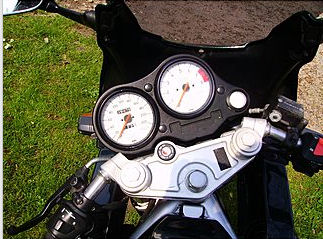This outdoor photograph features a unique, motorized bike that diverges from the standard motorcycle design. The bike is situated on a grassy terrain, with a dirt section visible in the top-right corner. The image captures partial handlebars and a stainless steel main section at the center. There are two circular gauges, though their functions are indiscernible. At the top left of the frame, an extension with a mirror is apparent, hinting at a potential rearview component. However, on closer inspection, elements of the setup such as these mirrors and gauges suggest that this might be a specialized piece of equipment, possibly related to photography. The additional attachments may indicate this is a custom rig, perhaps incorporating light meters or other photographic tools.